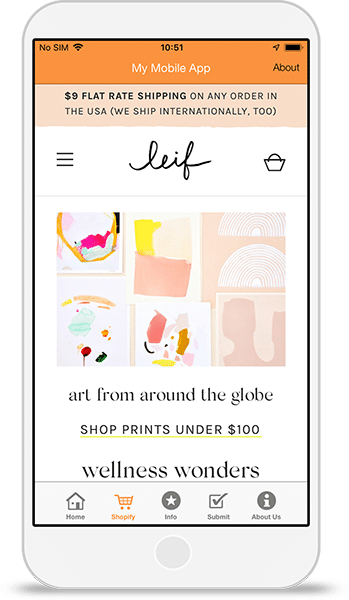A screenshot of a mobile application interface. The top header is an orange bar labeled "My Mobile App," which appears to be clickable. Directly beneath it is a lighter orange bar announcing, "$9 flat rate shipping on any order in the US. We ship internationally too." Below these announcements is a white area featuring a hamburger menu icon, script text that reads "LEIF," and an icon resembling a shopping bag. The main content area displays a piece of non-representational modern art with the caption, "Art from around the globe." Underneath the artwork is the text, "Shop prints under $100," with an underline indicating it is likely a hyperlink. At the bottom, the section labeled "Wellness Wonders" is presented, followed by a gray bar with a slightly darker dividing line. This bar includes icons labeled Home, Shopify, Info, Submit, and About Us.